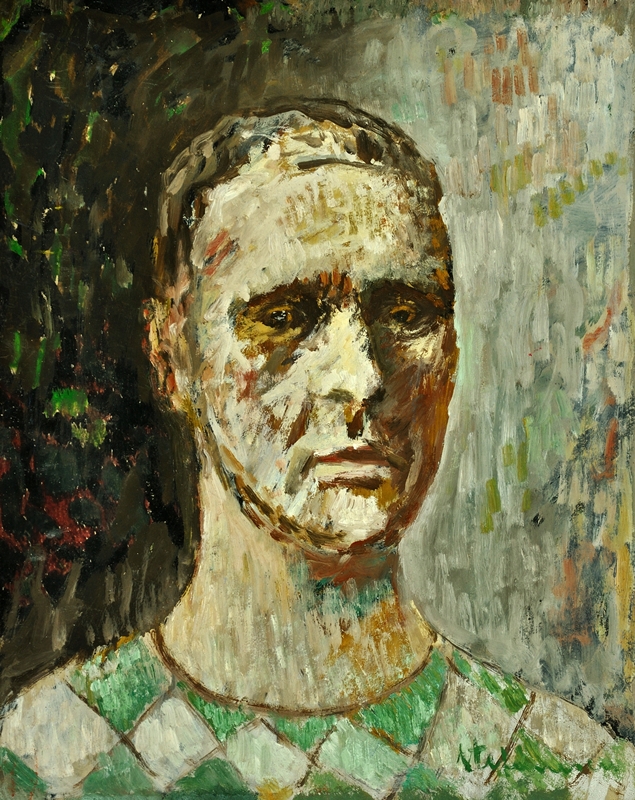This image features an impressionistic oil painting of a man's head and shoulders. The man's skin is pale, with notably splotchy areas of even lighter paint, adding a sense of rawness and emotional depth to the portrait. His short, Zuckerberg-like hair frames a somber face staring slightly off to the right, giving a melancholic impression. His attire is a checkered shirt with alternating rows of green and white, adding a subtle, yet contrasting detail. The background is distinctly divided: dark, greenish-brown tones on the left and lighter, cream and greenish-gray hues on the right. This division enhances the painting's impressionistic style, characterized by small, short brush strokes. The painter's signature is subtly placed in the bottom right corner, adding a finishing touch to this intimate, evocative portrait.